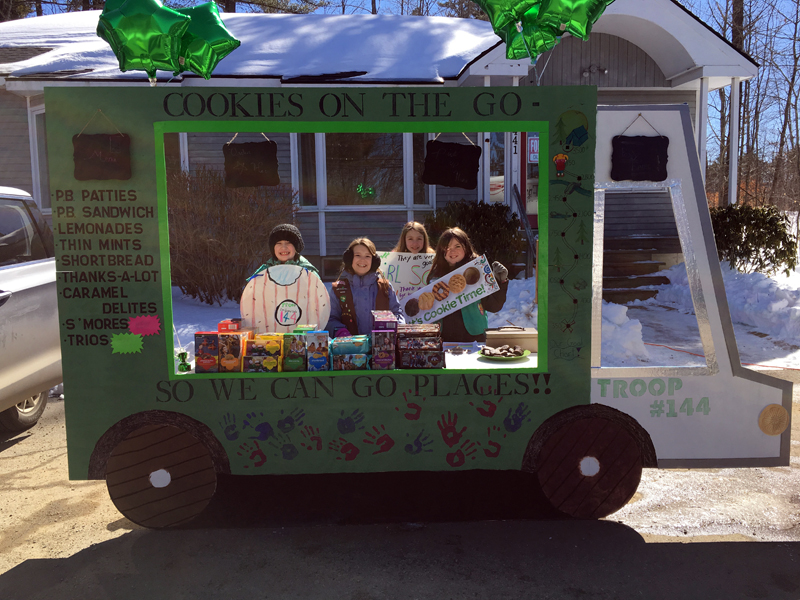Captured in a serene winter setting, this daytime photograph showcases a picturesque scene of freshly fallen snow in front of a cozy house. The driveway and pathway have been meticulously shoveled, creating clear, welcoming paths amidst the white blanket of snow that covers the ground and dusts the roof. Leafless trees, stripped bare by the season, frame the scene, enhancing the stark beauty of winter.

In the foreground, a charming tableau unfolds at a makeshift station where a green truck made from a cardboard cutout stands prominently. This delightful display features enthusiastic children selling Girl Scout cookies, adding a touch of warmth and cheer to the wintry day. The cardboard cutout is creatively adorned with the slogan "Cookies on the Go – So We Can Go Places," inviting passersby to indulge in the seasonal treat. This image captures the essence of community spirit and the simple joys of a snowy winter day.